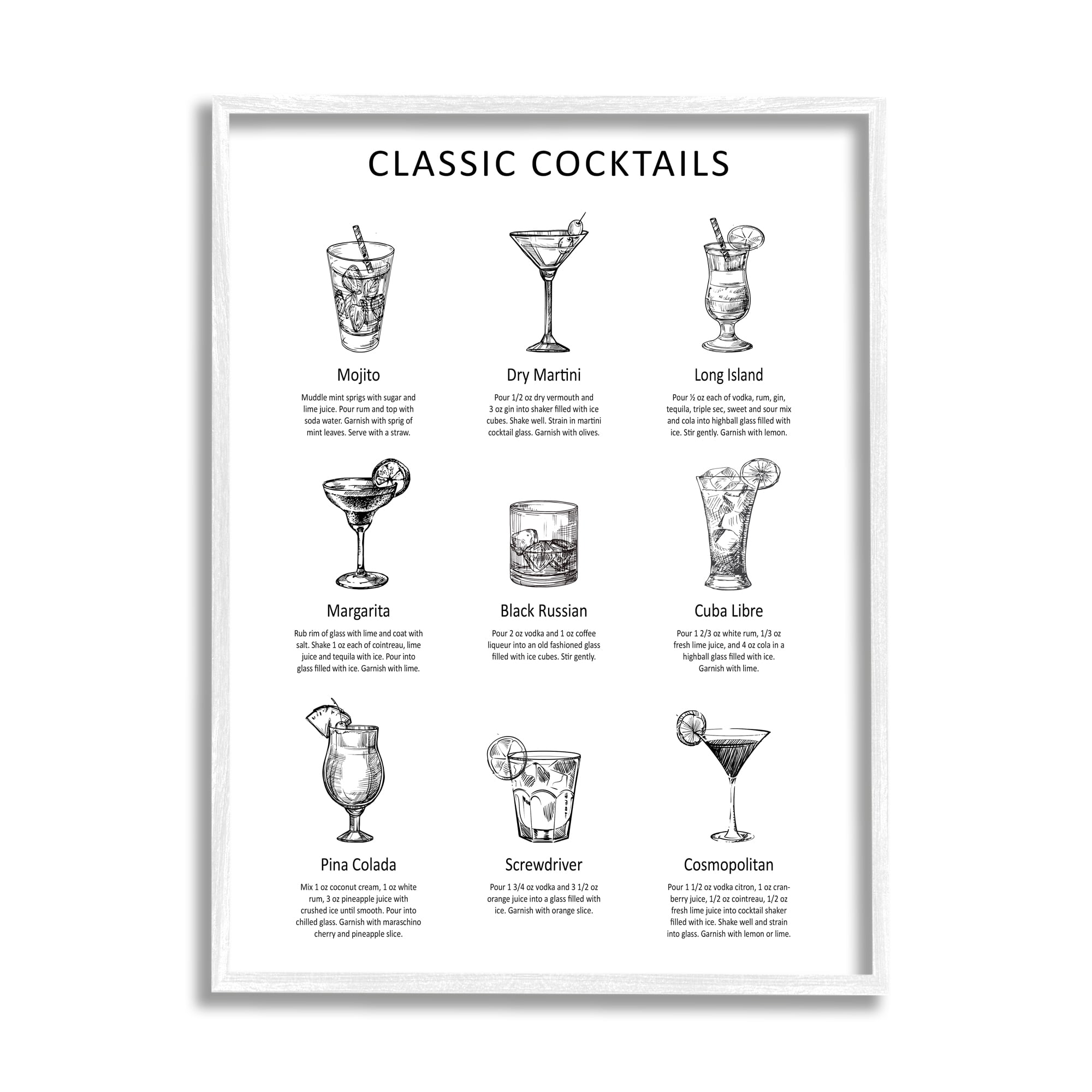The image features a framed picture with a thin, white border. Inside the frame, there's a white background adorned with intricate black pen drawings. At the top, the title "Classic Cocktails" is prominently displayed. Below it, the artwork is organized into three rows, each containing three detailed illustrations of cocktails, accompanied by unreadable descriptions.

In the top row:
1. A "Mojito" is illustrated with a cocktail glass, though the detailed description remains illegible.
2. A "Dry Martini" is depicted with a classic martini glass and an olive garnish.
3. A "Long Island Iced Tea" is shown with a tall glass, straw, and an unspecified slice of citrus.

In the middle row:
1. A "Margarita" appears in a margarita glass, garnished with a citrus slice.
2. A "Black Russian" is represented by a simple glass filled with ice.
3. A "Cuba Libre" is illustrated as a tall glass with ice and a slice of citrus.

In the bottom row:
1. A "Pina Colada" is depicted in a glass featuring a slice of pineapple.
2. A "Screwdriver" is shown in a small glass, accompanied by a slice of citrus.
3. A "Cosmopolitan" is presented in a martini glass, also garnished with a slice of citrus.

The black-and-white nature of the drawings lends a classic, timeless feel to the depiction of these well-known cocktails.